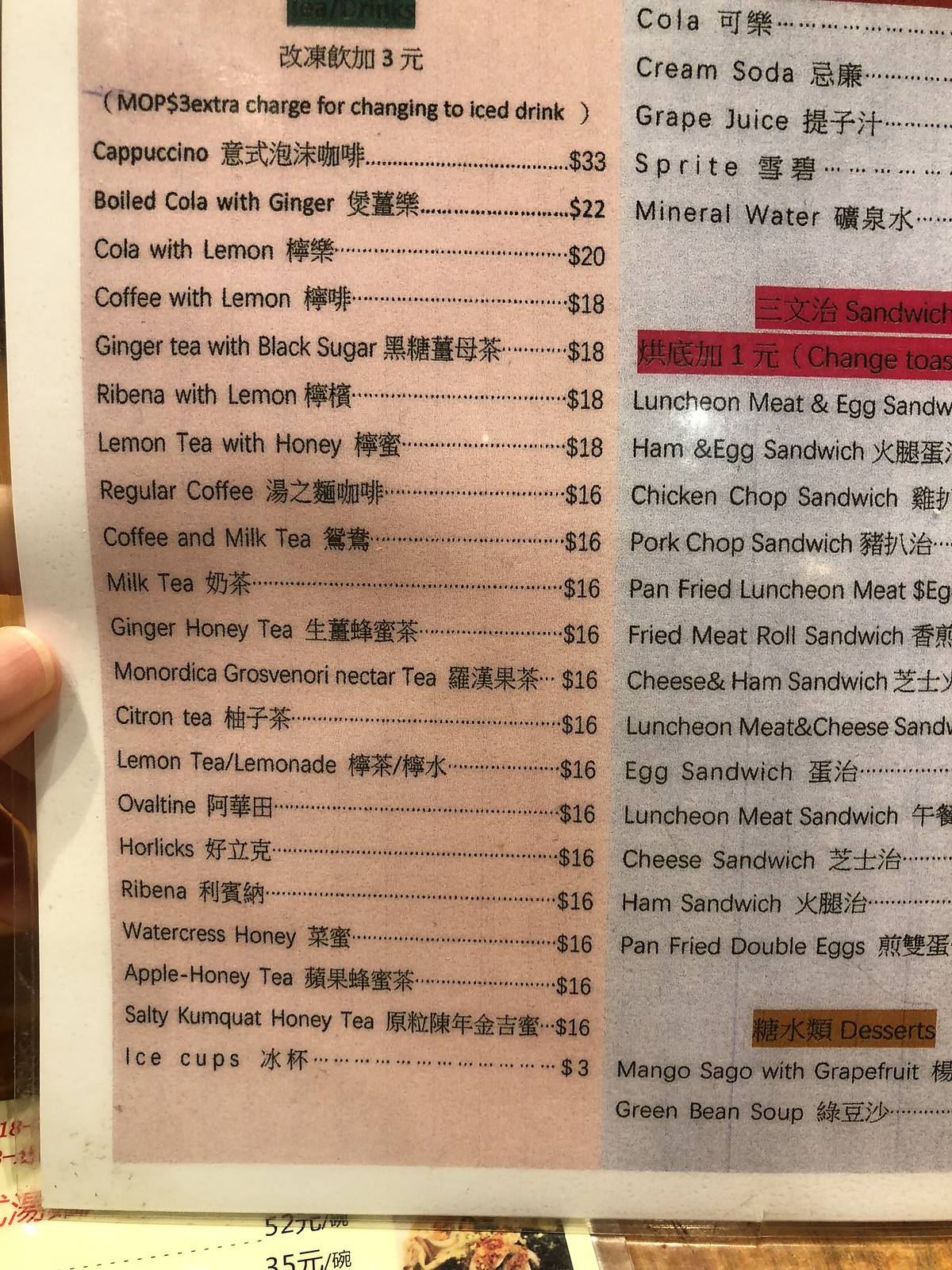A colorful menu is displayed on a table, accompanied by another menu sheet featuring a couple of images. The main menu has a pink section on one side and a blue section on the other. The extensive drink list includes various options such as iced beverages at an additional cost, cappuccino, boiled cola with ginger, cola with lemon, coffee with lemon, and ginger tea with black sugar. Other drinks offered are Ribena with lemon, lemon tea with honey, regular coffee, coffee with milk tea, milk tea, ginger honey tea, Monardica Grovis Nora nectar tea, citron tea, lemon tea, lemonade, Ovaltine, Harleks, Ribena, watercress honey, apple honey tea, salt tea, kumquat honey tea, and ice cups.

Additionally, the menu features a distinct section marked with a red cross, listing a variety of sandwiches such as luncheon meat and egg sandwich, and ham and egg sandwich, among others.

The juxtaposition of the pink and blue sections along with the diverse range of beverages and sandwiches gives an inviting and comprehensive view of the menu offerings.